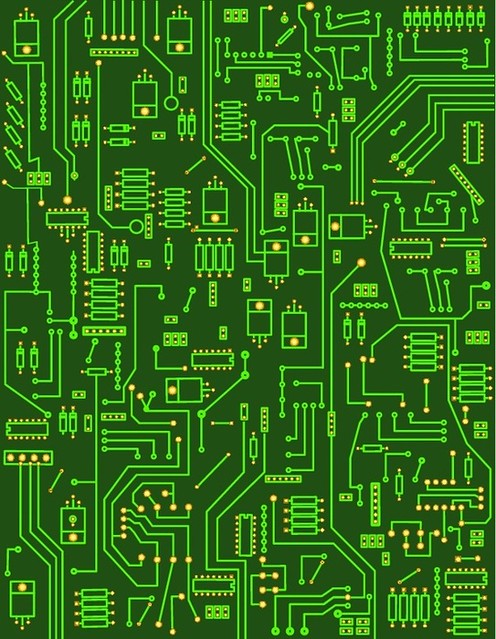The image depicts a highly detailed circuit board, showcasing an intricate network of electronic components and pathways. The background is a dark emerald green, densely populated with bright neon green circuit lines forming complex, maze-like patterns. Among these circuits are numerous small, golden spots that serve as connectors, giving the board a hint of vibrant yellow highlights. Various electronic components such as transistors, resistors, and other essential elements are visibly scattered throughout the board. Despite the lack of any text or labels, the board's design suggests it's a vital part of a larger electronic device, possibly a computer or other advanced machinery. The detailed layout of the circuits and components creates a visually striking image, emphasizing the intricate and essential nature of the technology within.